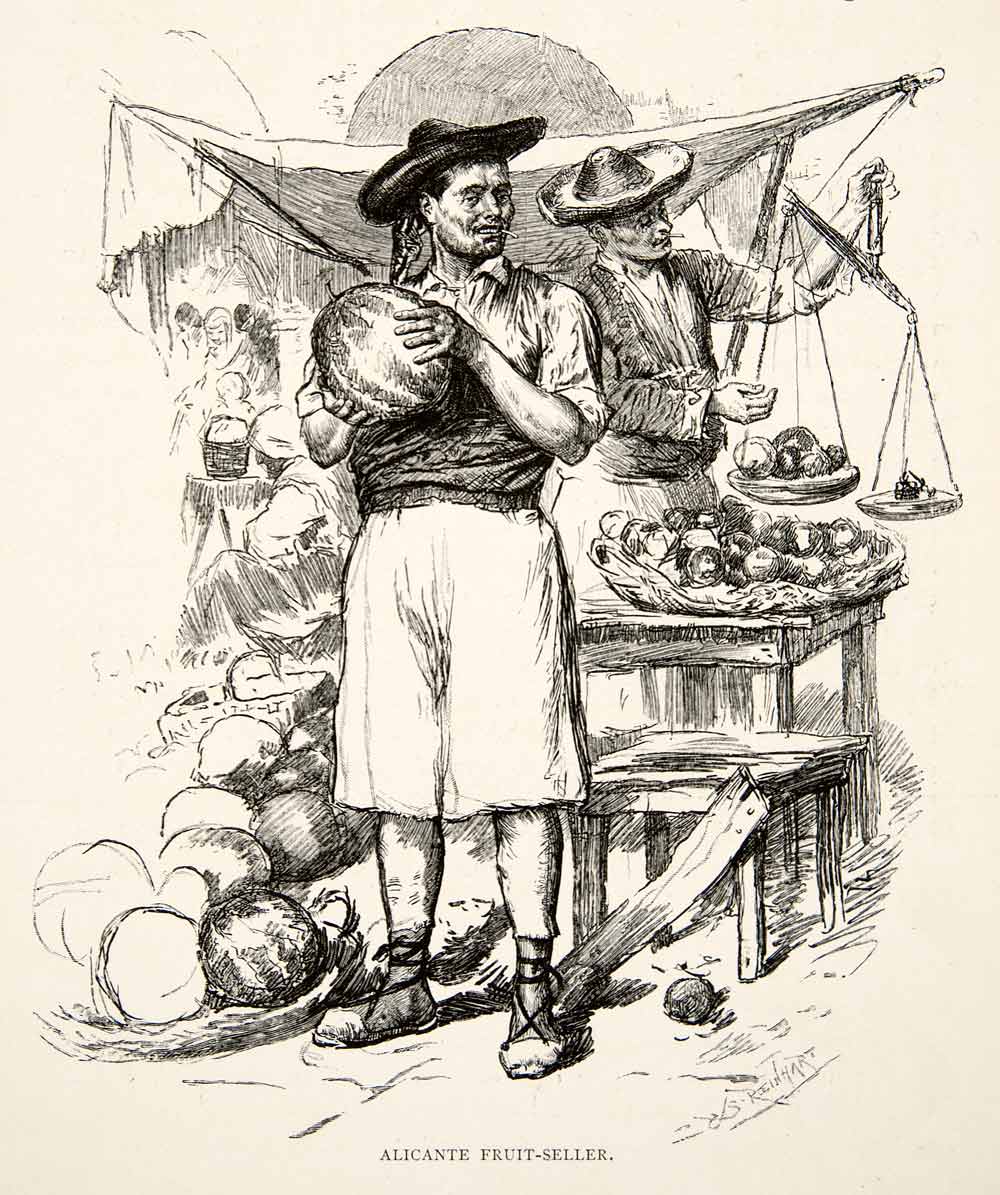This visually striking black and white line drawing, set on paper that appears to have a tinted pinkish or brownish hue, captures a bustling market scene titled "Alicante Fruit Seller." Central to the image are two South American men, readily identified by their traditional hats and attire. 

The man in the foreground, donning a black sombrero, is depicted in a rolled-up long-sleeve shirt and white baggy shorts that extend below his knees, along with sandals featuring ankle straps. He holds a watermelon, distinguishable by its unique lines and size, and he appears to be chewing on a cylindrical object, possibly a cigar or cigarette. 

Adjacent to him stands another man, also wearing a sombrero and engaging with a rustic scale that has two plates. This man is positioned next to a crude table loaded with a basket full of spherical fruits, likely apples. Melons are scattered on the ground beside them.

Further into the background, various figures, including women, can be seen shopping, contributing to the lively ambiance of the market. Underneath a canopy, more stalls brim with produce like cabbage, adding depth and context to the scene. The detailed depiction of the scale, the variety of fruits, and the interaction between the figures enriches the illustration, making it a vivid portrayal of a traditional market.